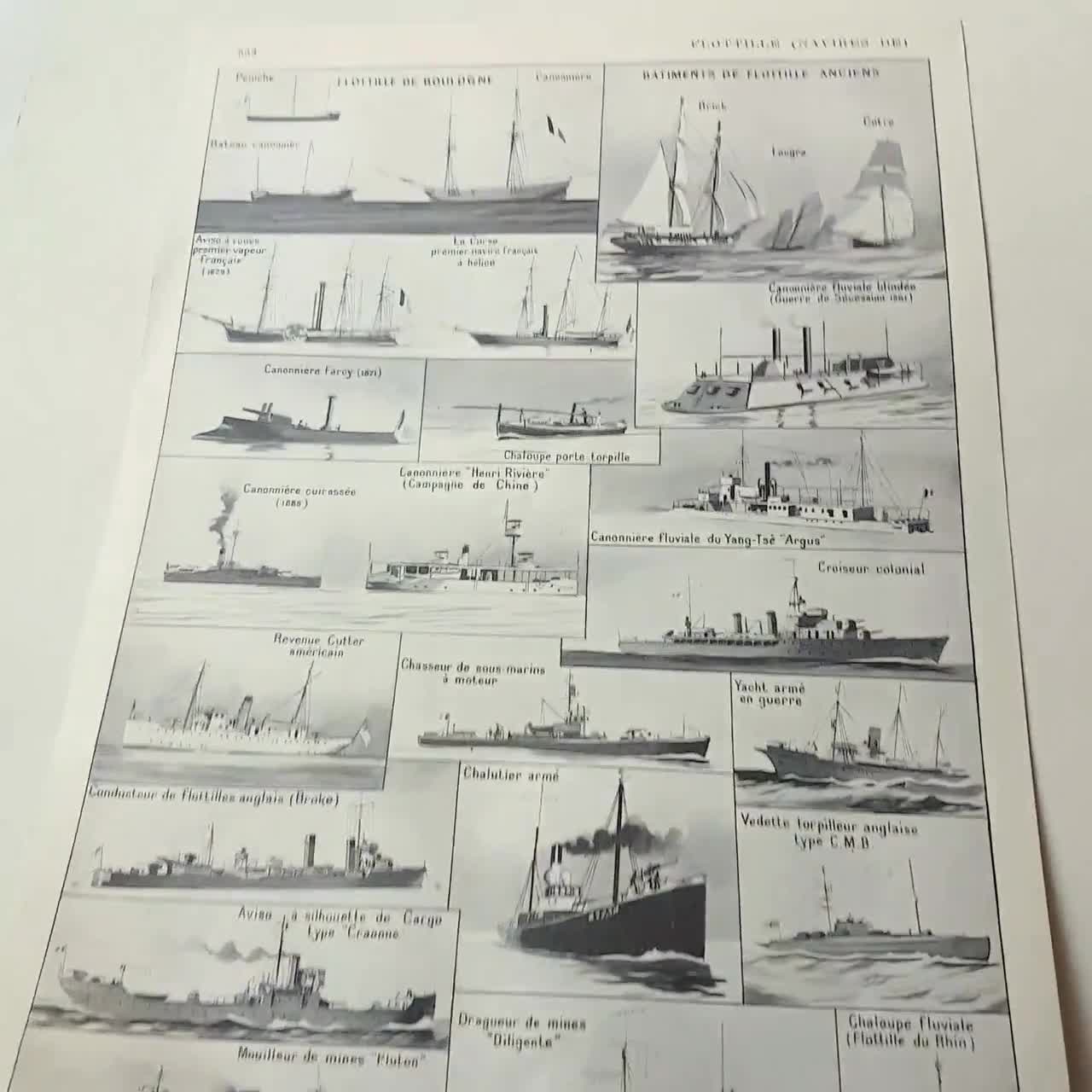The image depicts an old black-and-white poster or diagram showcasing a collage of approximately 20 to 23 boats. These vessels range from smaller wooden boats at the top, symbolizing historical styles, to more modern, military-style warships at the bottom, illustrating the progression of naval engineering through history. The ships are sketched in various angles and the entire image appears to be grayscale with no color. The poster likely includes descriptions next to the illustrations, but the text is in an unreadable foreign language, possibly French, making the exact details hard to decipher. The overall photograph of the poster is slightly blurry, with the upper part being brighter and more difficult to read. Additionally, there is a faint number, possibly 533, visible on the top left of the poster. Based on context, it appears to be depicting the evolution of French flotillas from the Age of Sail through steam-powered Ironsides to steel-hull modern warships.